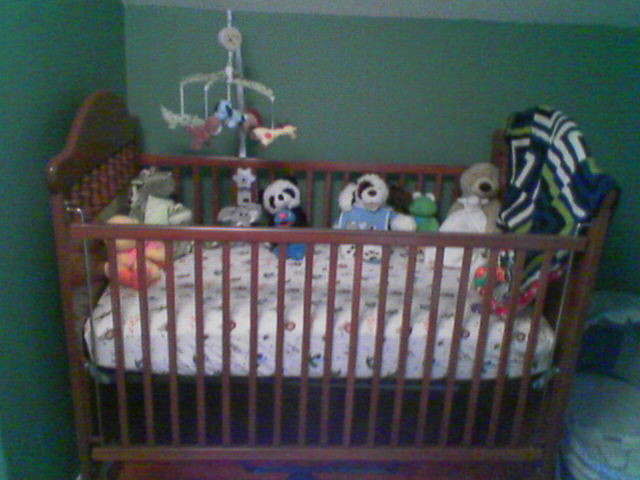In this photograph, which has a grainy and blurry quality indicative of being taken with an older camera, we see a baby's crib positioned in the corner of a room with dark green painted walls. The crib is made of a dark reddish-brown wood with bars on both sides that can be raised and lowered. Inside the crib, there's a white mattress adorned with a polka dot-type pattern, though the exact designs are indistinguishable. Several stuffed animals line the interior, including a small black-and-white panda, a white dog with brown patches, a green frog, and a light gray bear with a black nose. Additionally, a blanket with white, blue, and green stripes is draped over the right side of the crib. Dangling above the crib is a decorative mobile featuring various stuffed animals arranged in a circular motion, providing a playful element to the scene.